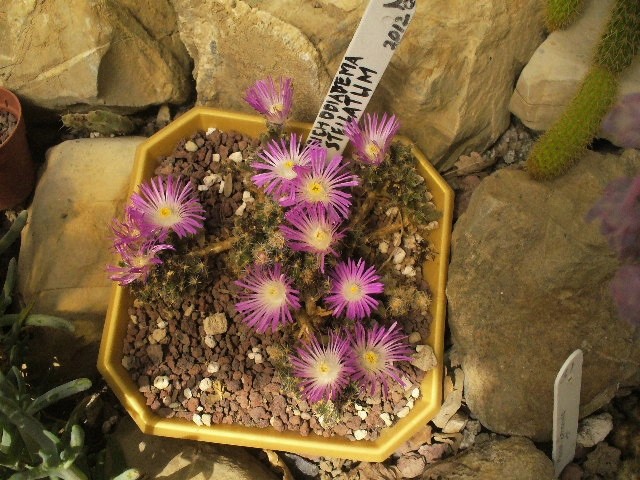The image depicts a yellow plastic container filled with dirt, housing several green, round cacti. These cacti are adorned with vibrant purple flowers that have white centers and yellow stamens. Inside the container, gray rocks or gravel are also visible, further supporting the plants. A white rectangular label protrudes from the top of the pot, with the text "Rhychodyma stellatum, 2012" inscribed on it. The container is surrounded by numerous large gray rocks, and to the right, there is a cucumber-shaped, light green cylindrical cactus resting on one of the rocks.